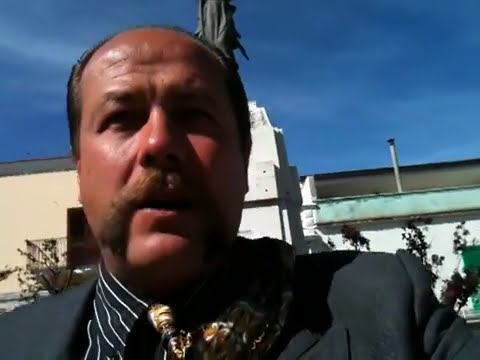The image is a close-up photograph of a middle-aged Caucasian man with reddish, sunburned skin. He has a distinctive brown handlebar mustache and short brown hair that is thinning at the top. The man is wearing a gray blazer over a black and white collared shirt with vertical stripes, along with a gold-patterned tie. The photograph appears to be a selfie, likely taken outdoors during the day. In the background, there is a partly cloudy blue sky, a white concrete building with some mint green trim, an exhaust pipe, and a grayish-green statue that is mostly obscured by the man's head. To his right, over his shoulder, a portion of a crepe-colored building is visible, and there are also vines growing up one of the structures. The overall scene is outdoors and captures the detailed texture of the man's face and attire, as well as the architectural elements behind him.